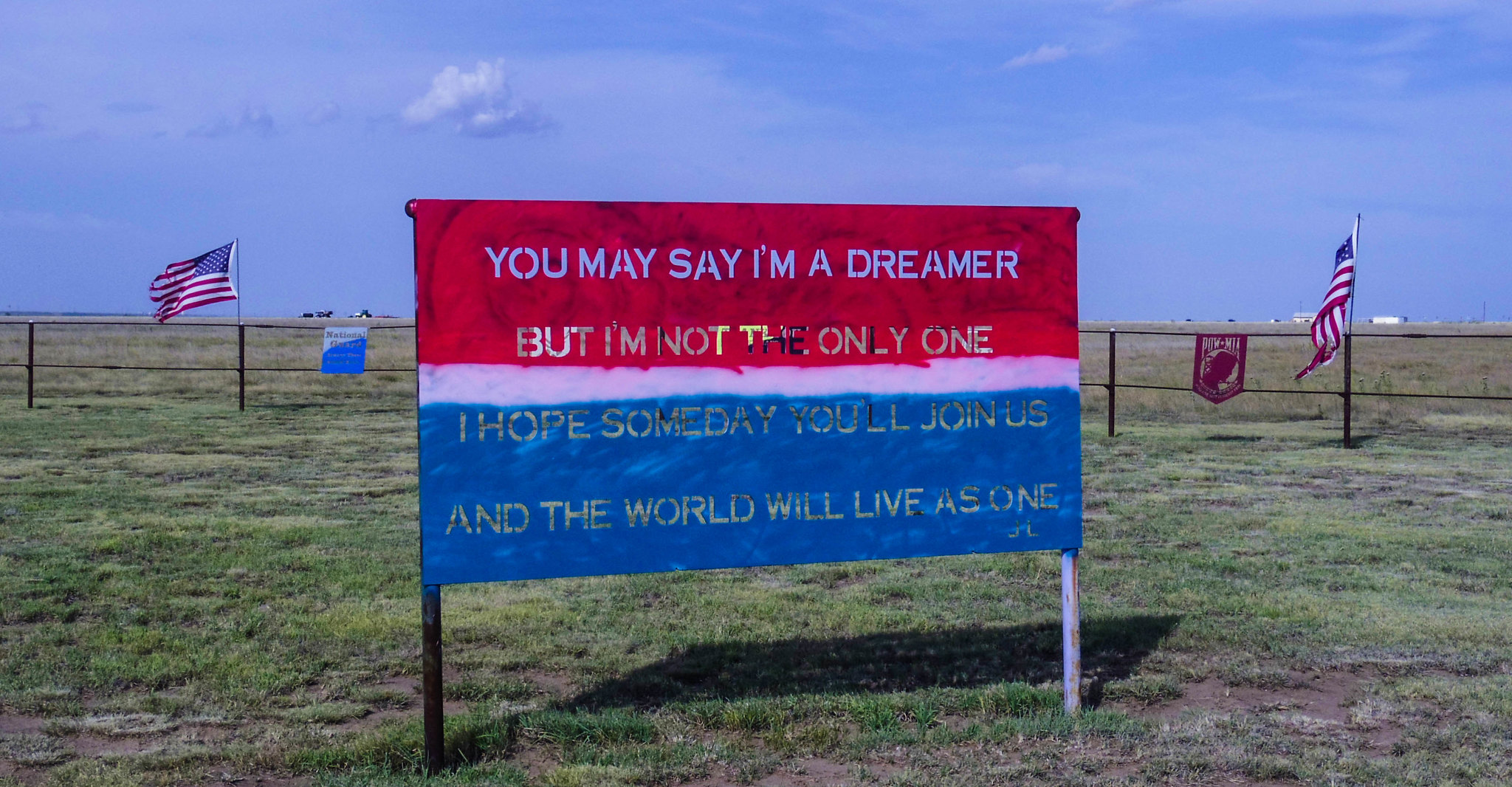The image is a color photo presented in landscape orientation, showcasing an outdoor scene in a well-maintained, large green field. Dominating the center of the photo is a banner mounted on two posts, positioned closer to the bottom half of the image. The banner features red, white, and blue horizontal stripes, with the central white stripe being quite narrow. 

The red portion at the top displays the quote in white lettering: "You may say I'm a dreamer, but I'm not the only one." Below the white stripe, the blue section carries the continuation of the quote, also in white letters: "I hope someday you'll join us, and the world will live as one." The letters seem slightly transparent, as if stamped onto the banner. 

In the background, a black fence adorned with a "Palmea" sign runs horizontally, with U.S. flags flying on both sides, mounted on the fence posts. The grass beyond the fence is slightly taller, and beyond that, buildings are faintly visible but indistinct. The upper half of the image is filled with blue sky and clouds, enhancing the photograph's sense of realism. The scene may depict either private or public property.